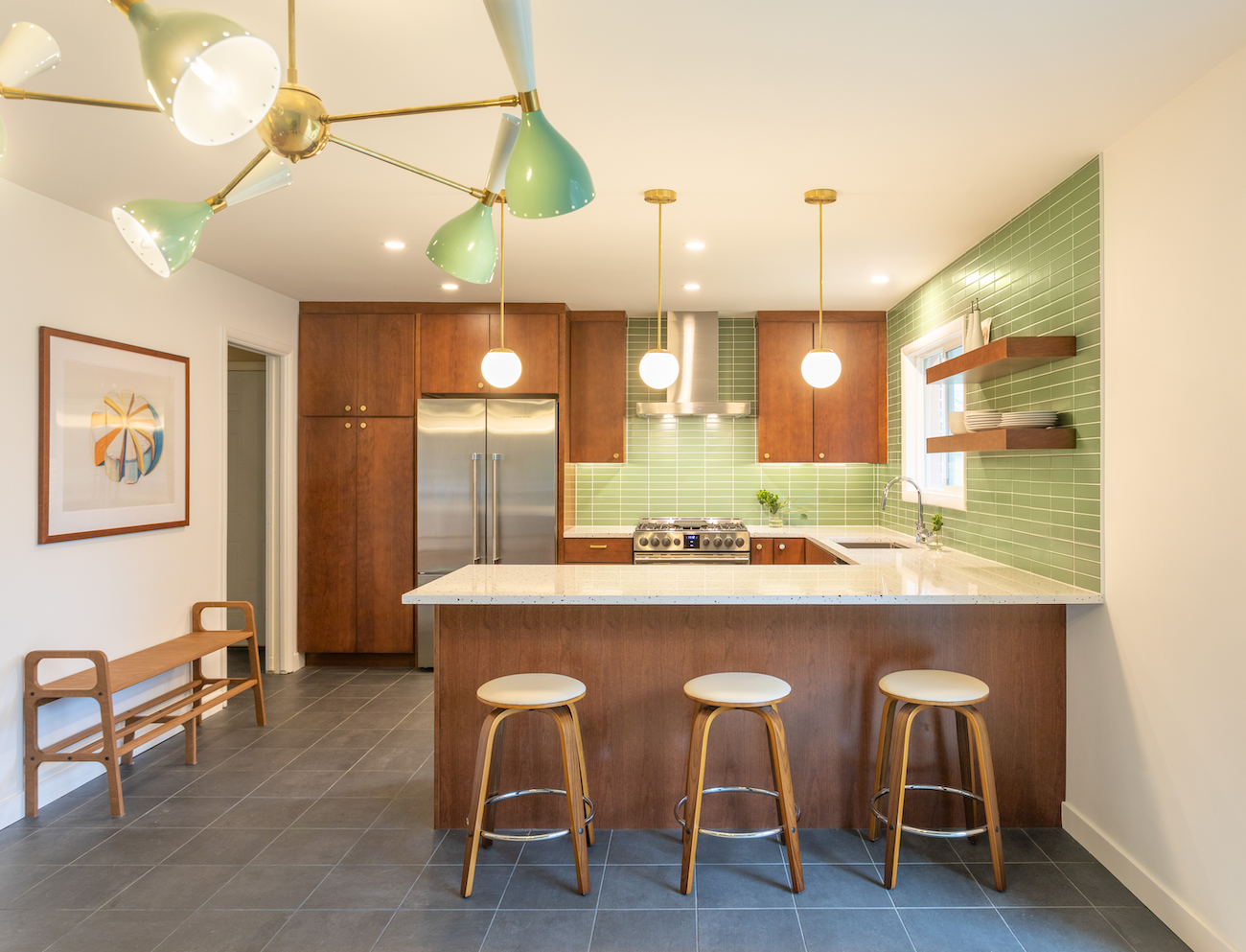The photograph captures a mid-century modern style kitchen. Dominating the back wall is a stainless steel refrigerator flanked by floor-to-ceiling dark brown cabinets. Adjacent to the fridge is a stainless steel oven with a matching range, set against a striking light green subway tile backsplash that extends to the ceiling and wraps around the kitchen. The left and right walls are painted white, enhancing the room's brightness. A framed picture depicting a circular object sliced into eight pieces, resembling a cake, adorns the left wall, below which a wooden bench is positioned. Floating wooden shelves are visible on the right wall. The ceiling is adorned with an interesting chandelier that features light green elements matching the tile backsplash. Three globe-like lamps hang down from gold rods above a white granite countertop that extends into a bar area. Here, three stools with white tops and wooden legs are neatly arranged. The flooring contrasts the space with a subtle gray hue, complementing the kitchen's cohesive design.